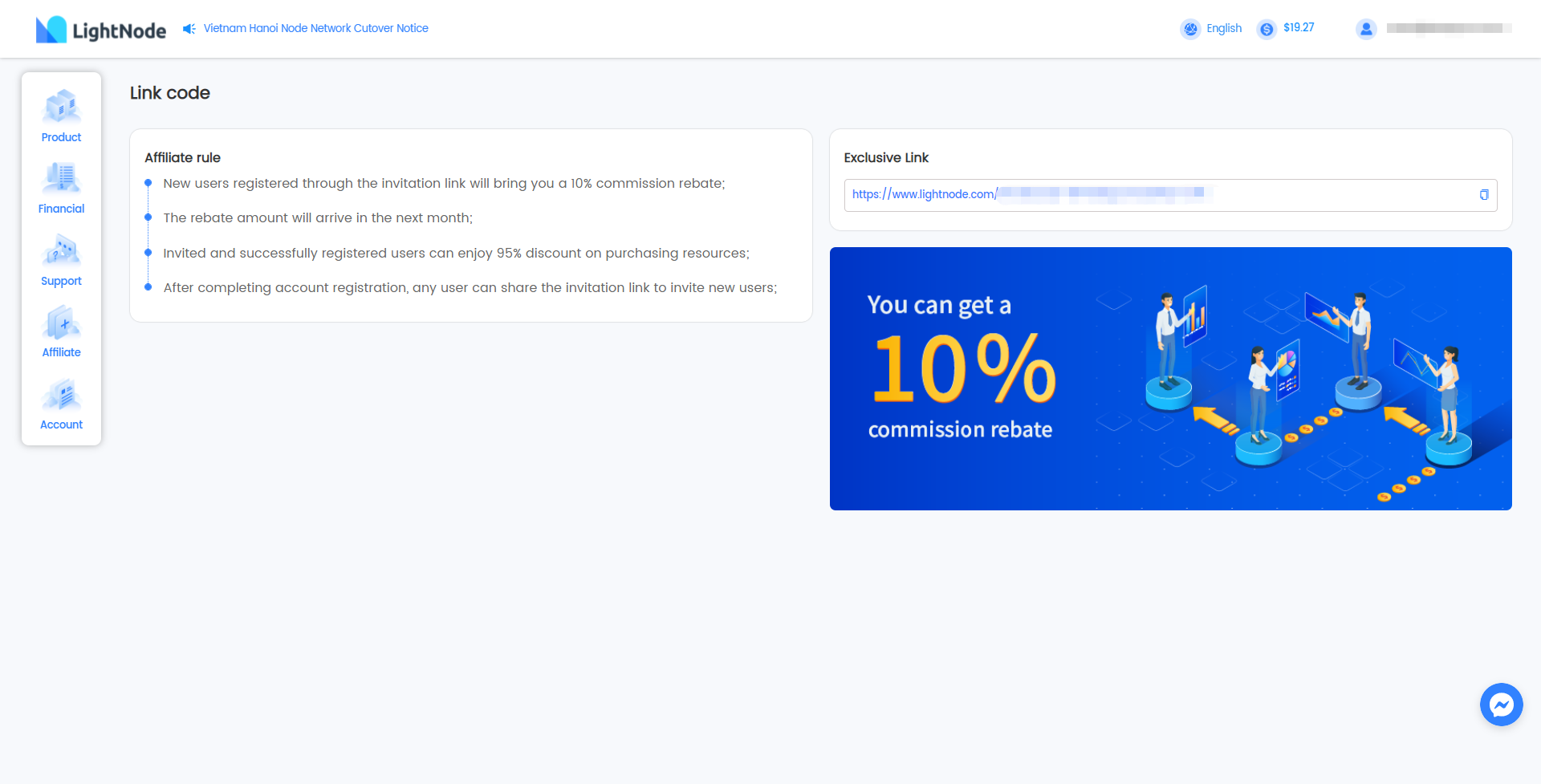The screenshot depicts a profile interface with a color scheme consisting of light blue, dark blue, and light node elements. The text is in English, and the profile icon is accompanied by a gray-scratched-out name for privacy. There are several features listed including a "link code" and an "affiliate rule," which mentions that new users registering through the provided invitation link will generate a 10% commission rebate for the referrer. This rebate amount is scheduled to arrive in the following month. 

On the far left side of the interface, a navigation menu includes options such as "Product," "Financial," "Support," "Affiliate," and "Account." The section also offers an "Exclusive Link," displaying the first portion of the website's address in blue, while the second part is blurred with a white line overlay. Highlighted in yellow, the text reiterates the "10% commission rebate." Additionally, at the bottom of the screenshot, there is an image depicting four people.